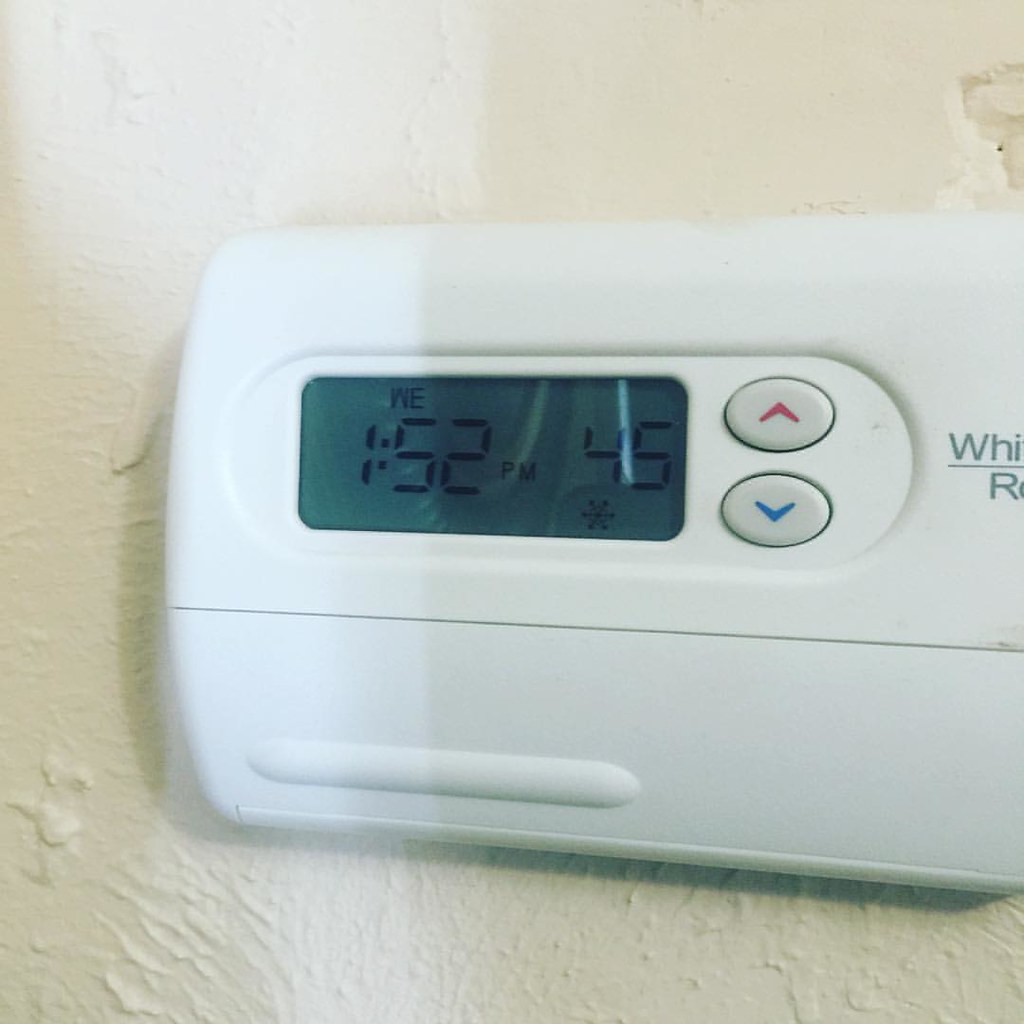An up-close shot of a digital thermostat mounted on a textured white wall, often found on ceilings, resembling the stippled pattern created by a dragged mop. The wall features light streaks that gently fall from the top left corner, tapering towards the center, and shine across the left side of the thermostat before fading out of view.

In the top right corner of the image, there's a noticeable chip missing from the wall, exposing more white underneath. The thermostat itself is prominently centered but positioned slightly to the right, stretching horizontally across two-thirds of the image and vertically leaving a couple of inches of wall space above and below it.

The thermostat face is divided by a central black line, demarcating the display from the controls. The top portion, beginning from the right, features the black lettering "WHI" atop a line, followed by another "R". Below this, two small gray round buttons sit, the upper one marked with a red arrow and the lower with a blue arrow. These are likely temperature adjustment controls. To the left of the buttons, the digital screen displays the temperature "152," an abbreviation "WE," and "45", with a small circle beneath the "4" containing a snowflake symbol, indicating a cooling mode.

The bottom-left corner of the thermostat has a slightly raised piece, possibly a latch for accessing internal components like batteries. The overall image captures the functional and worn-in aesthetic of this household device.